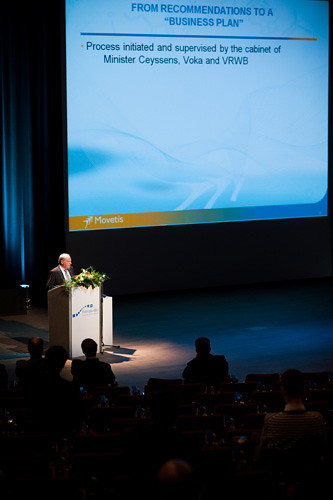In this image, a man is delivering a presentation on a stage. He is positioned behind a podium, dressed in a suit and tie, speaking towards the right side of the frame. The podium is adorned with a white poster featuring blue writing that is not fully legible, and a bouquet of flowers is also present atop it. Behind the man, a large white screen dominates the background, displaying the text "From Recommendations to a Business Plan" at the top, followed by a long blue line spanning from left to right. Beneath this line, the text reads, "Process Initiated and Supervised by the Cabinet of Minister Cessners, VOCA, and VRWB," although some letters are difficult to discern. Framing the screen are curtains along the back of the stage. The lower portion of the image is darkened, revealing an audience seated in rows of chairs, attentively watching the presentation. The setting suggests a formal seminar or conference room.